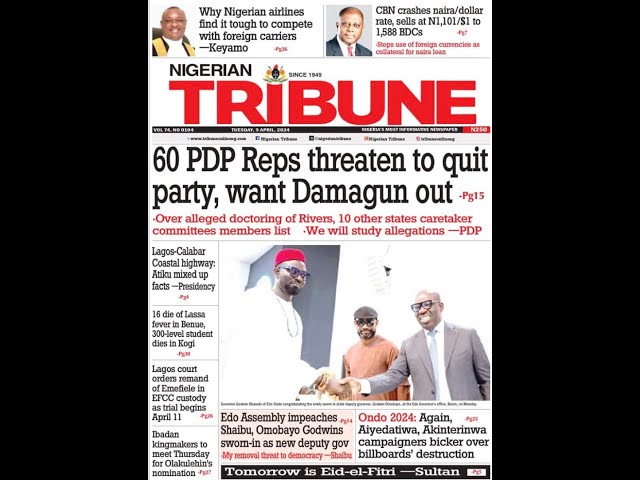This is the front page of the Nigerian Tribune newspaper, featuring a bold red "Tribune" header. The primary headline reads, "60 PDP Reps Threaten to Quit Party, Want Damagun Out," with further details on page 15 about alleged doctorings of caretaker committee members lists from Rivers and ten other states. The main image shows three African men, presumably of Nigerian descent, dressed in formal attire and all wearing glasses; two of the men are shaking hands, suggesting a conference setting. Additional headlines include: "Why Nigerian Airlines Find It Tough to Compete with Foreign Carriers" on the top left, and "CBN Crashes Naira-Dollar Rate, Sells at N1101/$ to 1588 BDCs" on the top right. The page is also dotted with various blurbs directing readers to other articles inside the newspaper.